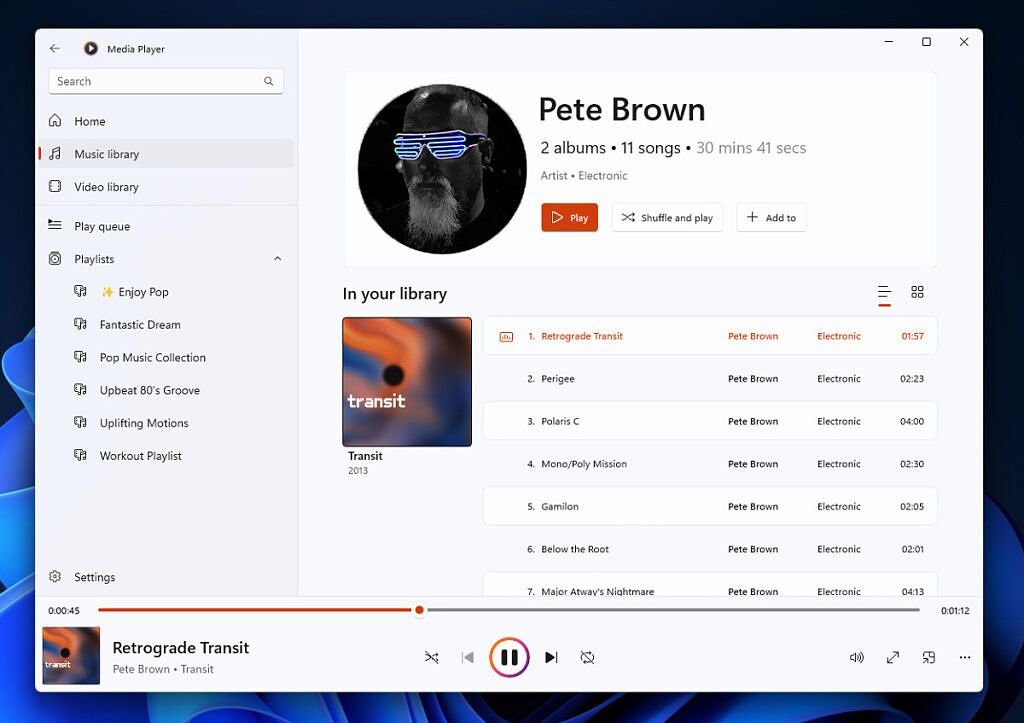The screenshot captures a desktop, dominated by a grayscale media player interface that covers most of the dark-themed background. The desktop wallpaper appears mostly black with intricate, wavy blue patterns flanking the sides and bottom edges. 

The media player displayed centrally is in various shades of gray. It features essential controls such as the back arrow, a search box, and the media player's logo. The main menu offers navigation options: Home, Music Library, Video Library, Play Queue, and Playlist. Under the Playlist section, there are several subcategories including "Enjoy Pop," "Fantastic Dream," "Pop Music Collection," "Upbeat 80s Groove," "Uplifting Motions," and "Workout Playlist."

The highlighted user profile showcases the artist Pete Brown, depicted with a circular avatar of a man wearing neon glasses in grayscale. The profile details include two albums encompassing 11 songs with a total playtime of 30 minutes and 41 seconds. Pete Brown is identified as an electronic music artist. The interface includes an orange "Play" button, a white "Shuffle and Play" button, and a "+ Add To" option.

In the user’s library, the album "Transit, Transit" is visible along with a playlist associated with Pete Brown. Additional controls at the bottom of the media player include a pause button, left and right track selectors, volume control, expand screen option, and a cloud icon.